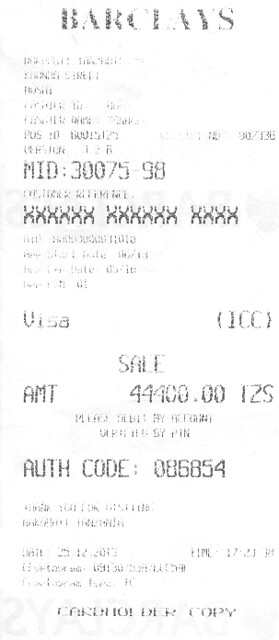A blurry and difficult-to-read receipt is prominently displayed in this photo. The receipt appears to be sealed, with a white background and black text. The top of the receipt is labeled with "Barclays." Immediately below this, there is some unreadable text. Further down, it lists "MID 30075-98," followed by multiple rows of 'X's and additional text that is obscured. In a clearer section, it states "Visa Sale AMT 44400.00125" and below this, the words "off code 086854" are visible. There is more unreadable text beneath, and at the very bottom, the phrase "Cardholder Copy" is printed.